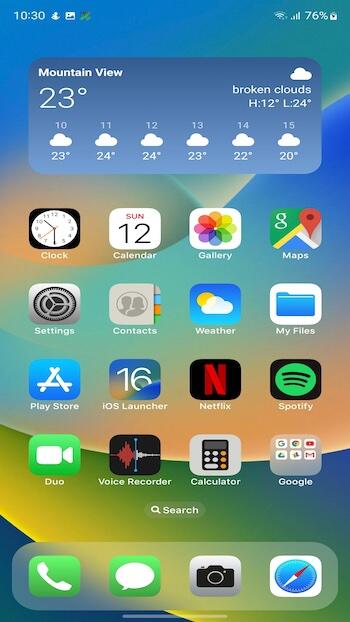This is a detailed screenshot from an iPhone's home screen at 10:30 AM. In the top-left corner of the screen, the time is visible, along with three notification icons. The middle icon appears to be a screenshot or photo gallery notification, while the first and third icons are not identifiable. On the top-right corner, you can see the Wi-Fi signal, mobile data indicator, battery percentage at 76%, and a charging icon denoted by an electric bolt inside the battery icon.

The home screen features a weather widget at the top, showing the location as Mountain View with a temperature of 23 degrees. The weather condition is described as 'broken clouds,' and the high and low temperatures for the day are listed as 24 degrees and 12 degrees, respectively. The forecast for the upcoming days is as follows: 
- 10th: 22 degrees
- 11th: 24 degrees
- 12th: 24 degrees
- 13th: 23 degrees
- 14th: 22 degrees
- 15th: 20 degrees

The app layout on the home screen is organized from left to right and top to bottom as follows:
- First row: Clock, Calendar, Gallery, Maps
- Second row: Settings, Contacts, Weather, My Files
- Third row: Play Store, iOS Launcher, Netflix, Spotify
- Fourth row: Duo, Voice Recorder, Calculator, Google (with a collection of Google apps)

Below these apps, there is a search button, and under that are pinned apps, which include Contacts, Messages, Camera, and Safari.